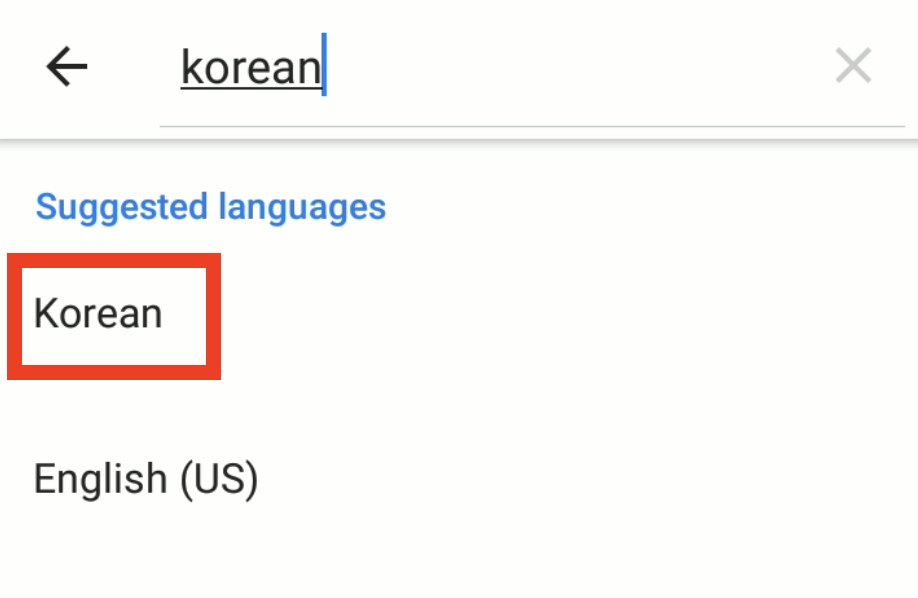This screenshot depicts a language selection interface. At the top of the screen, there is a search bar with the word "Korean" written in black, underlined, and immediately followed by a stationary blue cursor. To the top-left of "Korean" is a back arrow, and to the top-right is a small 'X' icon, suggesting these as navigation and close options, respectively.

Beneath the search bar, the interface displays a section titled "Suggested Languages" in blue text. Directly below this heading, "Korean" is prominently featured again in black text, enclosed within a box outlined in red. Following this, the text "English (US)" appears, also in black, listed as another language option. 

The entire section where the languages are listed is set against a clean, white background. Notably, the bottom edge of the search bar casts a subtle, gray drop shadow that appears slightly smudged.

Overall, the image is minimalistic, with little additional text or visual clutter against the predominantly white backdrop.